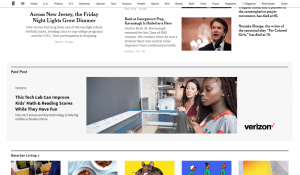**Caption:**

This image from a web page appears highly compressed, rendering the text difficult to read. The layout includes a white top background with a horizontal gray line about a quarter of an inch below. Above the line, on the left, are two black icons followed by small, illegible text that spans the width of the image, with 19 segments in total.

On the left side below the gray line, bold black text reads something about New Jersey and a Friday. Beneath this, there is a reference to "night lights" followed by additional details starting with "G" and "D." There are three very small lines of text below this part.

Centered in the image is bolded text spanning two lines, followed by five lines of smaller text, and a picture of a screaming man with black hair in a black suit. A chandelier is visible to his left. Next to the man are three lines of text and a gray bar at the bottom with two black words in the left corner, which are unreadable. Below this bar, three more lines of bolded text appear, followed by two smaller lines.

At the bottom-right is a picture featuring two girls: an African American girl on the right looking left, and a girl with black hair on the left looking forward. They seem to be examining something that resembles a printer. Adjacent to this image, the word "Verizon" is prominently displayed in bold black text with a red checkmark.

Five small images are lined up from left to right across the bottom edge of the image.